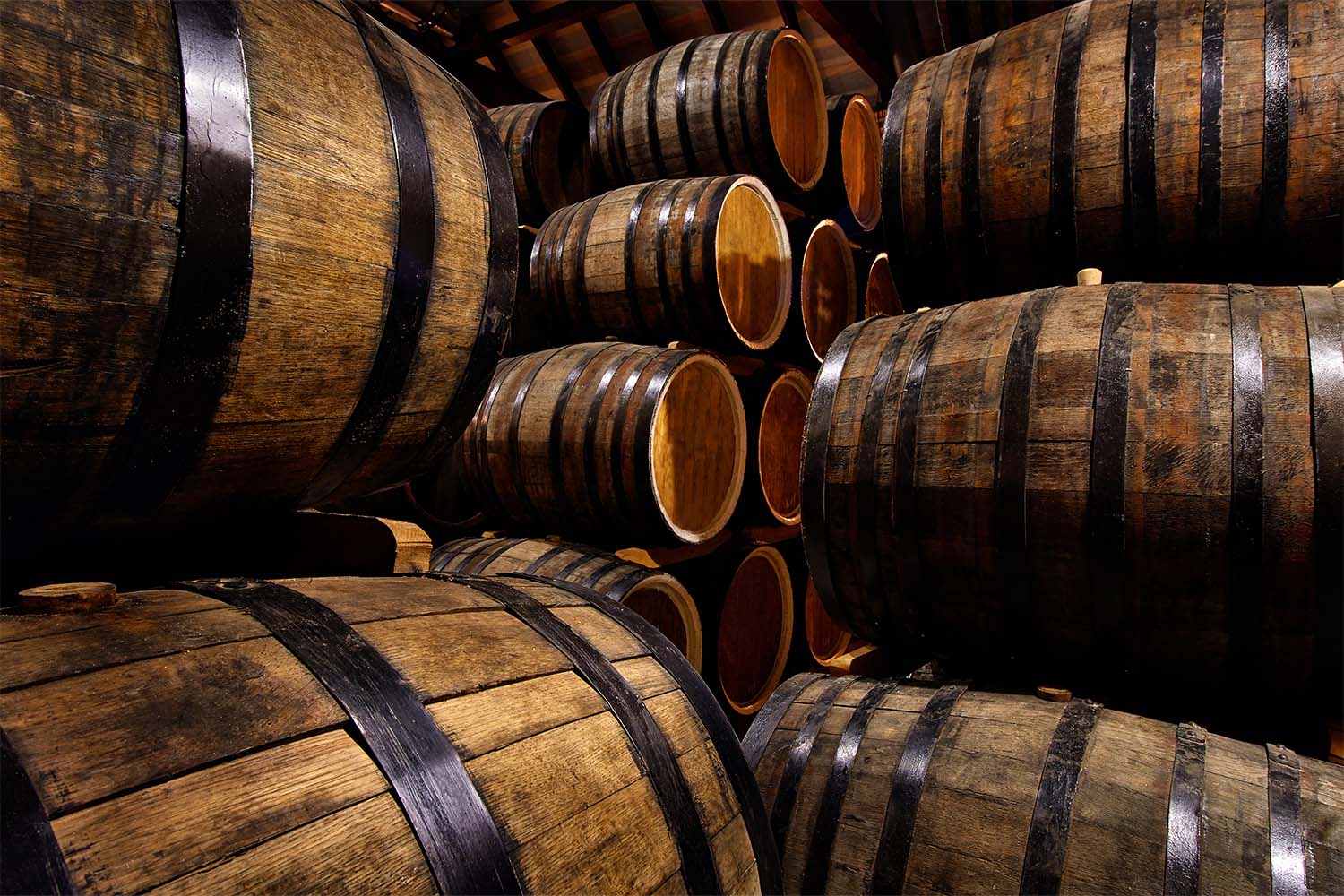This photograph captures a striking arrangement of large, dark brown wooden wine barrels stacked in a pyramid-like structure inside a spacious wooden building, likely a barn. The barrels, each adorned with seven to eight black metal bands, feature corks slightly protruding from three of the five prominently displayed in the foreground. These barrels are meticulously organized, with two placed on the left and three on the right, creating a symmetrical visual. Behind these five barrels, more are horizontally aligned, revealing their ends and extending deep into the background. The professional quality of the image highlights the rustic charm of the wooden interiors and the careful craftsmanship of the barrels, emphasizing their purpose in wine storage and maturation.